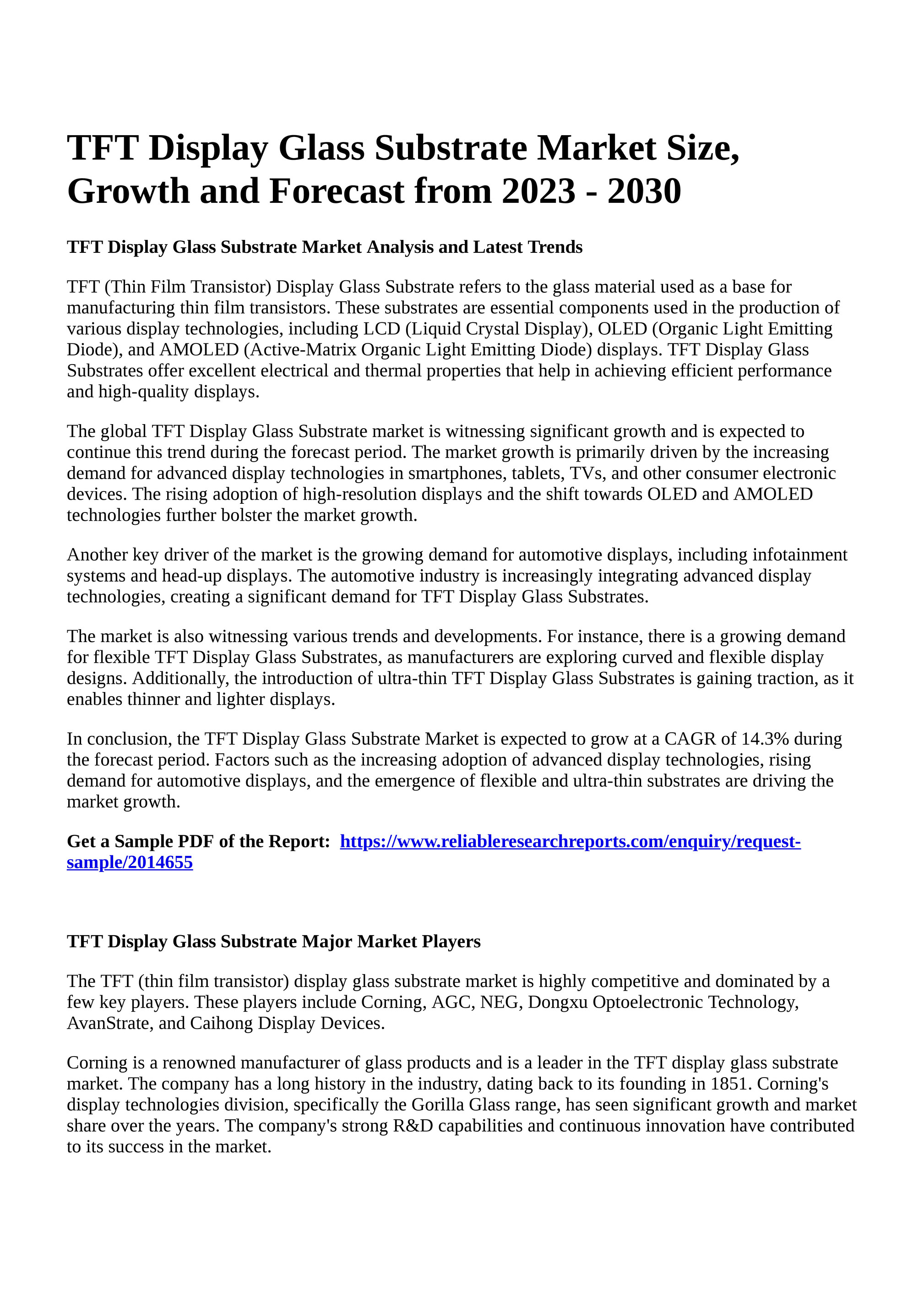The image features a detailed page of text on display against a plain white background with no border. At the top of the page, the bold black title reads "TFT Display Glass Substrate Market Size, Growth, and Forecast from 2023 to 2030." Directly beneath the title in slightly smaller, bold text, it states, "TFT Display Glass Substrate Market Analysis and Latest Trends." This is followed by several left-aligned paragraphs of black text. Below these paragraphs, there is a line prompting readers to "Get a Sample PDF of the Report," with a blue web address for further information. At the bottom of the page, there is another bold heading, "TFT Display Glass Substrate Major Market Players," followed by two more left-aligned paragraphs in regular black text. The content within these paragraphs likely mentions key industry players such as Corning and provides insights into the market trends, growth factors, and the increasing demand for advanced display technologies for devices like smartphones, tablets, and TVs.